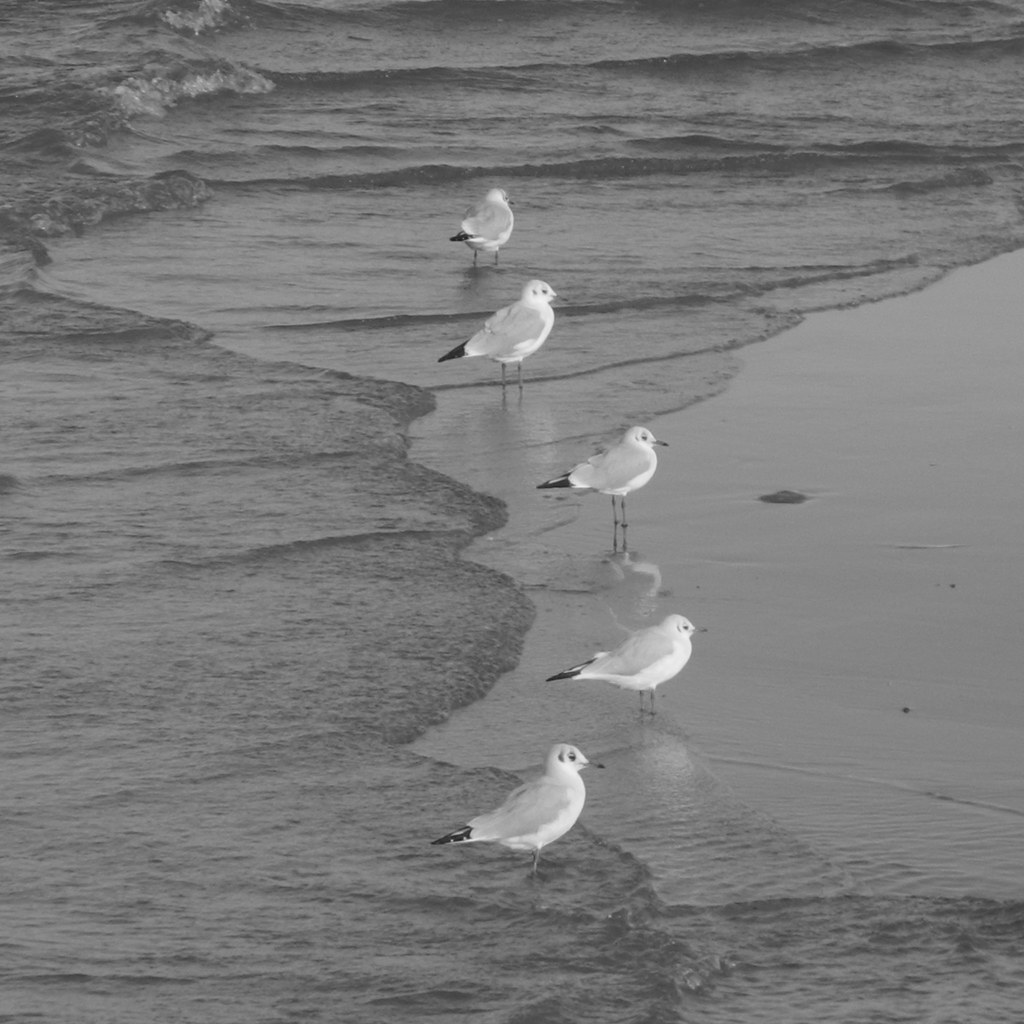This black and white image captures an intricate scene of five seagulls, or similar shorebirds, with predominantly white feathers and small black tails. They stand at various spots along a sandy shoreline, oriented from the bottom to the top of the frame and facing right. The shoreline itself is depicted with waves coming in from the left, creating a thin layer of water receding back into the ocean on the right. In the top-left corner, there is a subtle hint of either a sand dune or a rougher wave. The detailed birds are positioned side-by-side in the center, stretching vertically and almost covering the entire height of the image, giving a tranquil impression as they appear to be gazing out to sea.